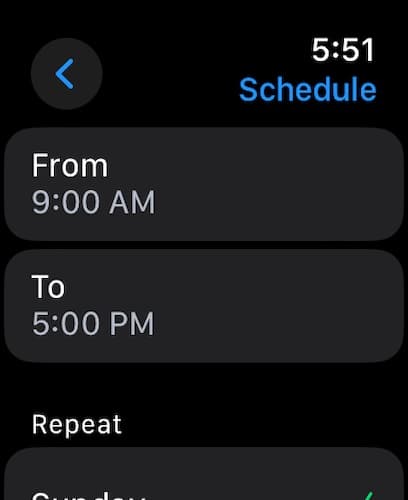This image appears to be a zoomed-in screenshot of a digital interface, possibly from a device with a small screen, such as a smartwatch or a compact app. The layout is in portrait orientation. On the upper left corner, there is a medium blue left arrow icon housed within a dark grey circle. The overall background of the application is a sleek black. 

In the upper right, the time is displayed as "5:51" without specifying AM or PM. Below the time, the word "Schedule" is prominently shown in blue text. 

Following this, there are three rounded rectangular cards spanning the width of the screenshot. The first card lists an event starting at 9 AM, while the second card indicates an event at 5 PM. 

Beneath these, there is another card, but before it, the word "Repeat" is displayed in white letters outside the card's boundary. This last card has truncated text, making it difficult to read, though a fragment of a green icon is visible in the lower right corner. The visual design includes notably large buttons, suggesting the interface is tailored for easy readability and interaction on a small screen device.